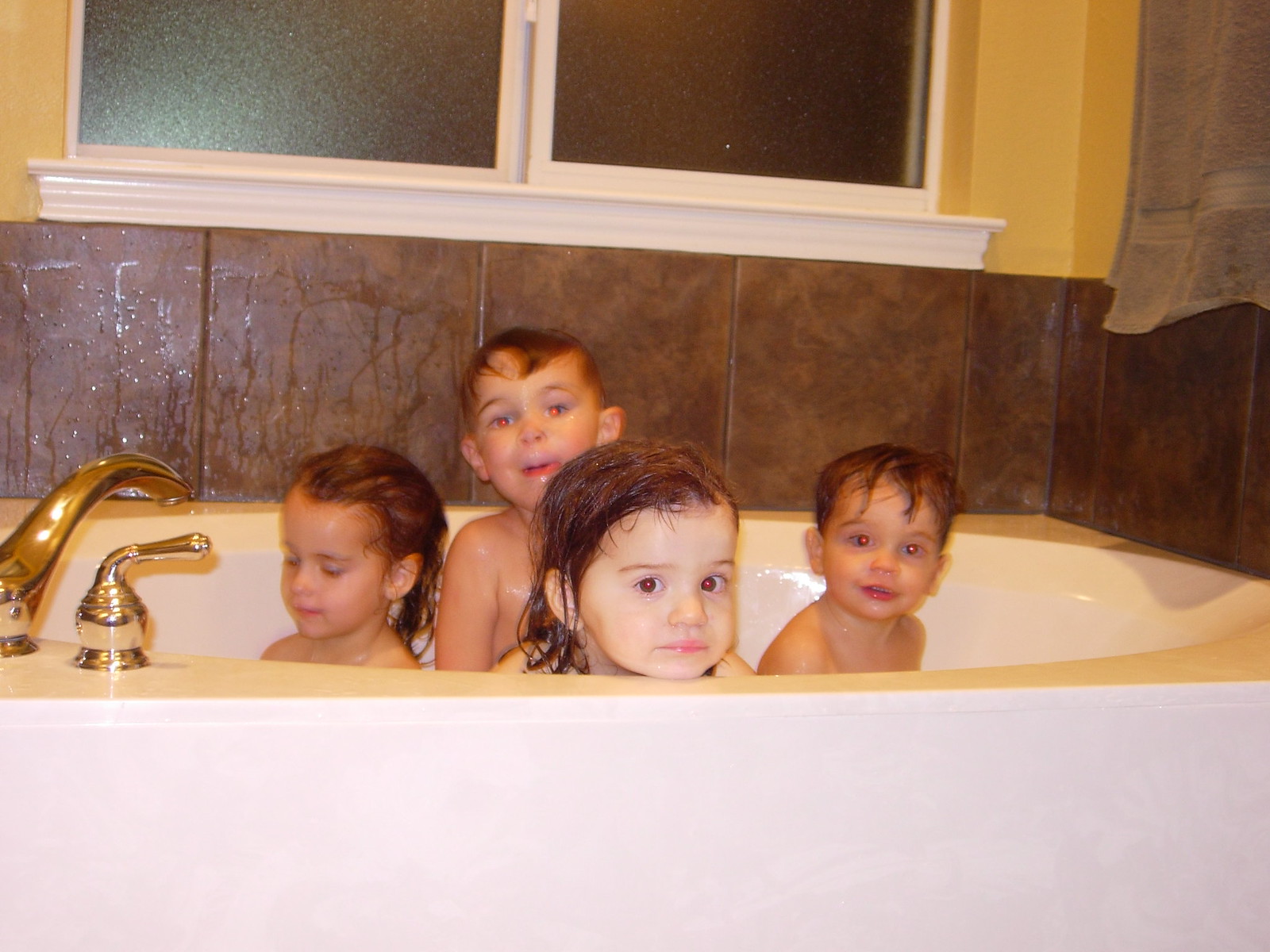In this charming family photograph, four young children are gathered together in a bright white, oval-shaped bathtub that exudes a touch of luxury with its gold taps and handles. The children, presumed to be two girls with long hair and two boys with short hair, are captured in various candid moments—three looking directly at the camera, their eyes appearing red due to the flash, while one looks down. One little girl is adorably resting her chin on the edge of the tub. The backdrop features large, brown ceramic tiles and a window above the bath with a frosted privacy screen and a white frame. The walls surrounding the window are a muted yellow-brown color, and a towel hangs neatly to the right. The overall scene is endearing, with a mix of vintage charm and warm household details.